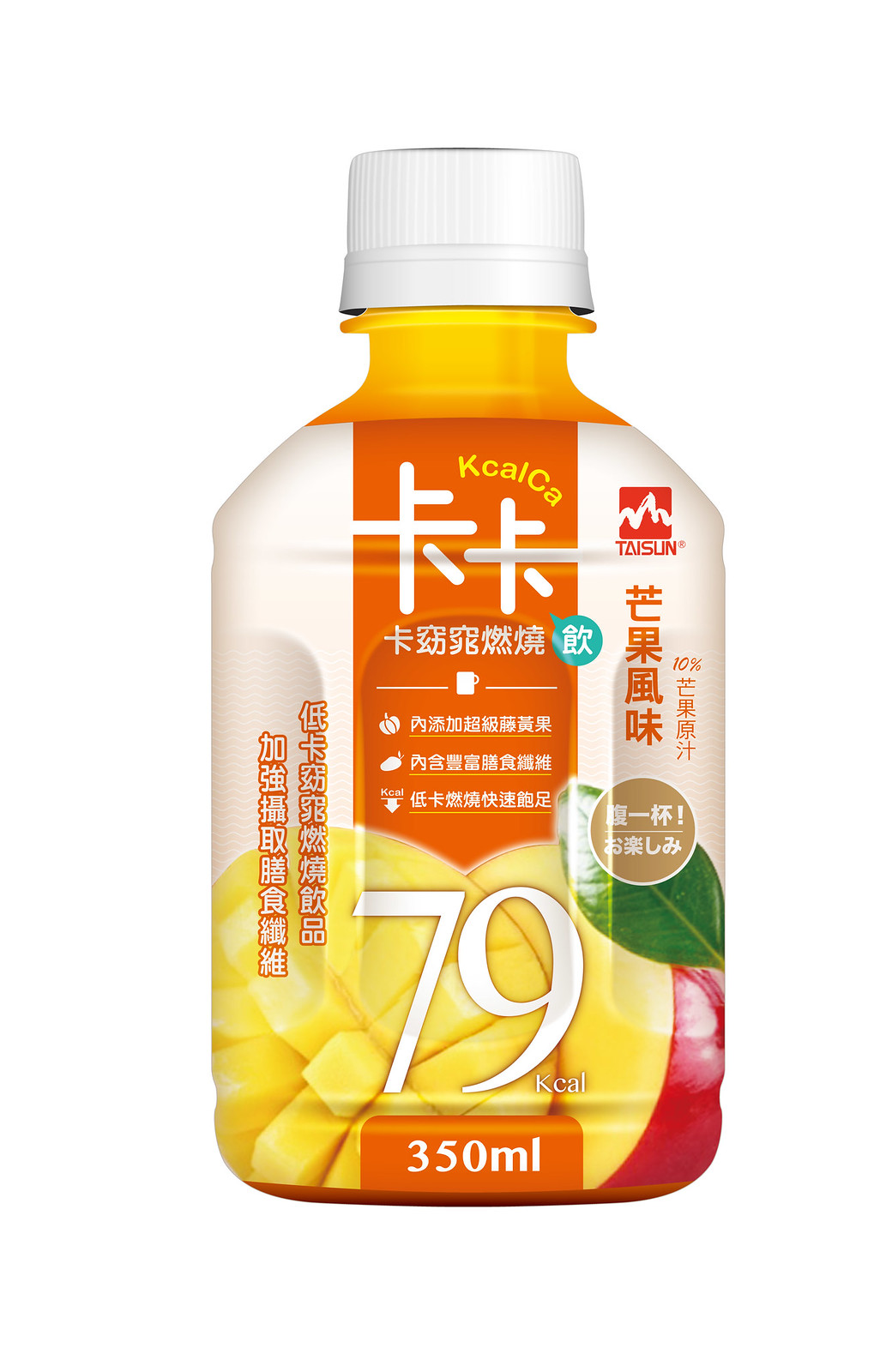This photograph features a short, wide bottle on a completely white background. The bottle is orange with a white twist-off cap, resembling a mouthwash bottle in shape. It has a plastic wrap adorned with intricate details and text, predominantly in Chinese. Prominently displayed on the bottle is a large "79" in white letters, indicating 79 calories (K-C-A-L), along with "350ML" inscribed in white text within an orange box. The wrap showcases vivid images of tropical fruits: two prominently displayed pineapples, a hedgehogged mango, and a diced mango, with glimpses of a small apple and its green leaf peeking behind them. The orange contents of the drink are visible within the clear plastic of the bottle, marking it as a nutritious and healthy fruit beverage.